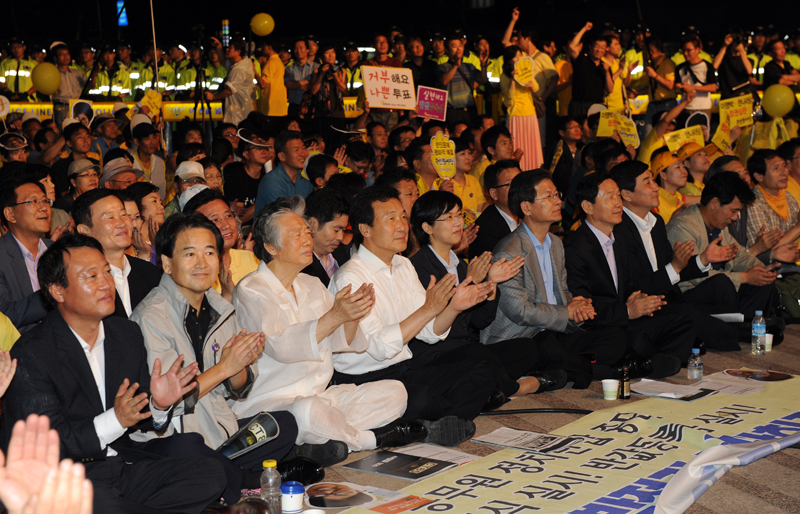The color photograph, taken in landscape orientation at night, captures a lively, celebratory scene dominated by a large crowd of Asian people. The background fades into darkness, accentuating the vibrant gathering illuminated in the foreground. At the center of the image, a semi-circle of individuals sits with their legs crossed, clapping and smiling as they look upwards towards the right top corner of the image. Behind them, a more animated group stands with arms raised, holding up posters and banners written in Korean text, along with yellow signs and balloons that add to the festive atmosphere.

Embedded at the feet of the seated individuals is a white, curved banner with text in Korean, contributing to the organized display. The realism of the photograph captures details such as the highlighter green and reflective vests worn by individuals in the background, suggesting the presence of security personnel, possibly firemen or police officers, overseeing the event. Overall, the image portrays a dynamic and celebratory night scene, filled with joy and communal spirit.